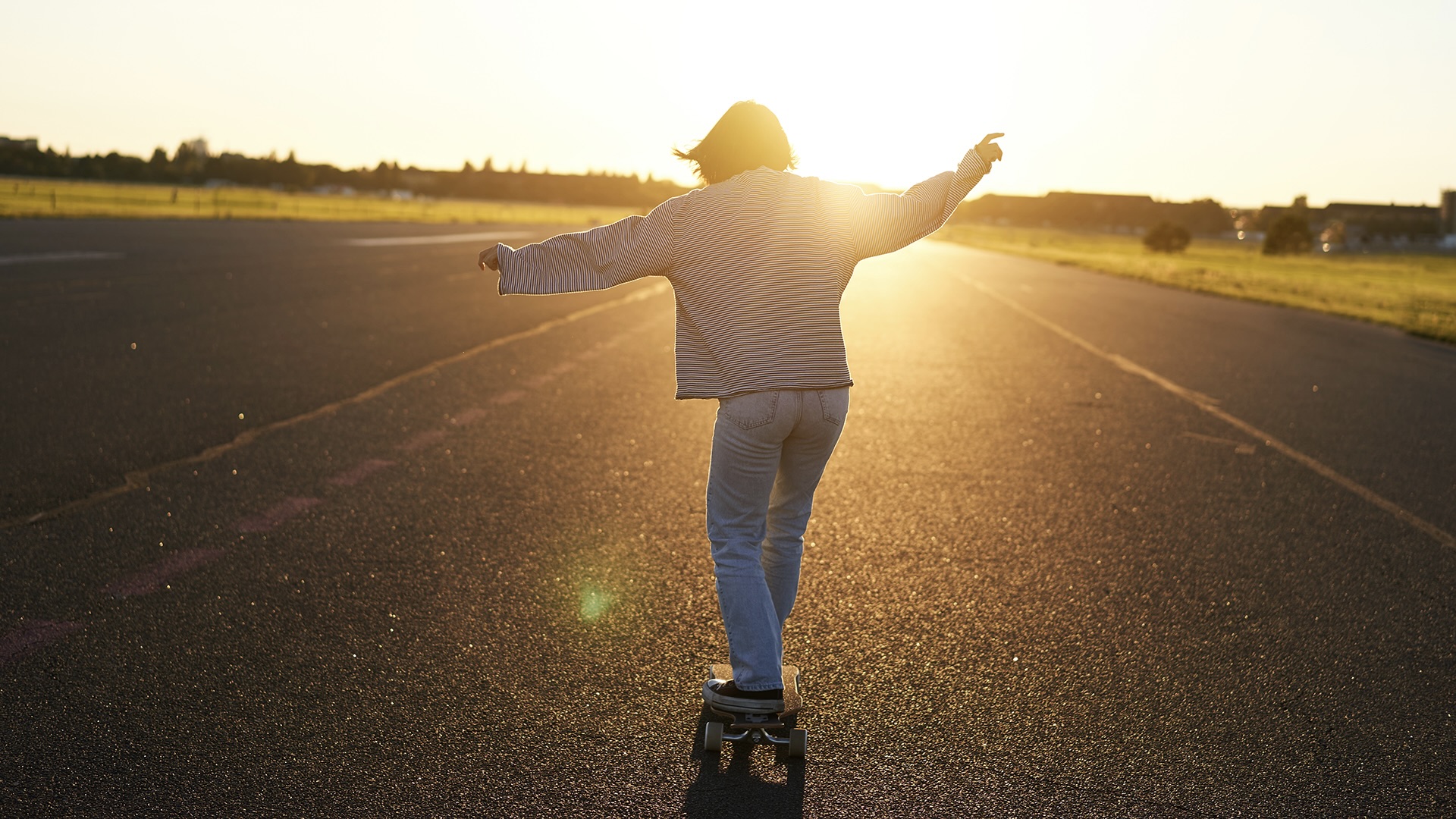The image depicts a girl with short dark hair skateboarding down an expansive, freshly paved, and deserted roadway that stretches towards the horizon where the sun is either rising or setting, casting a bright, blinding light. With her arms outstretched for balance, she wears a black and white striped long-sleeved shirt, light blue jeans, and skater shoes. Her hair flows with the motion, indicating she is moving rapidly. On either side of the road, distant greenery with trees and some scattered buildings can be seen, suggesting the scene is set on the edge of a suburb. The overall focus of the image is on her as she confidently coasts along the wide street, heading directly into the radiant horizon.